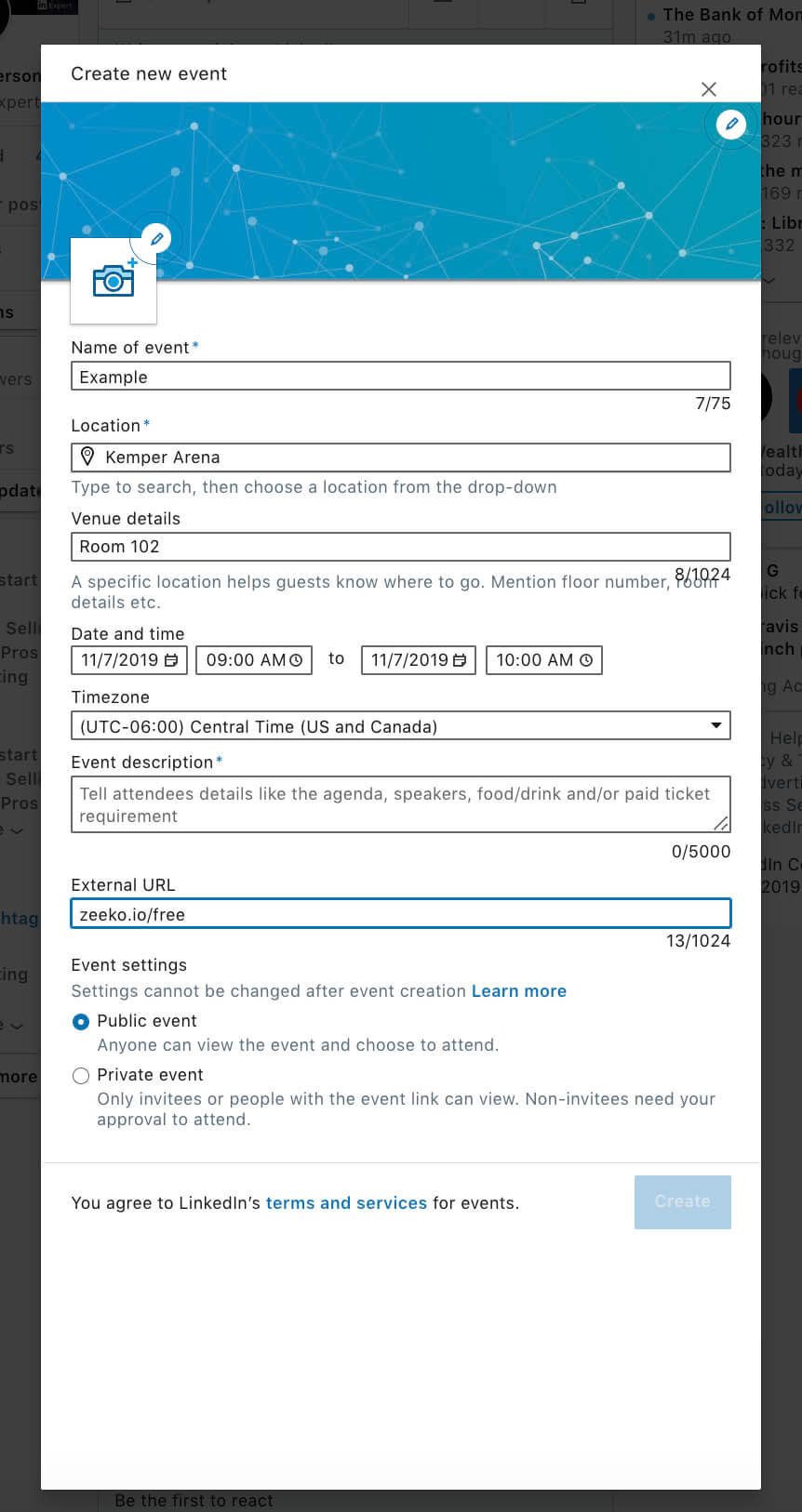A detailed descriptive caption for the image could be:

An electronic device, likely a tablet or smartphone, displays an application screen aimed at creating a new event. In the foreground is an interface with a title at the top that reads "Create New Event." A thick, banner-like bar stretches from left to right just below the title. This banner, featuring no text or profile picture, showcases a visually appealing constellation design with a gradient transitioning from blue to greenish-blue and interconnected stars or planets. 

Below the banner are fields for entering event details. The current information includes: event name (to be added), location set to "Kemper Arena," and venue details specifying "Room 102." The date is shown as either 07/11/2019 or 11/07/2019, based on regional formatting, with a start time of 9:00 AM and an end time of 10:00 AM. The selected time zone is Central Time (US & Canada).

The event description field encourages organizers to share key details like the agenda, speaker information, food and drink options, and ticket requirements. Additionally, there's a field for an external URL, which currently lists "zico.io/free." The event is set to be public. In the background, some indistinct text is visible, suggesting other open windows or documents on the device.